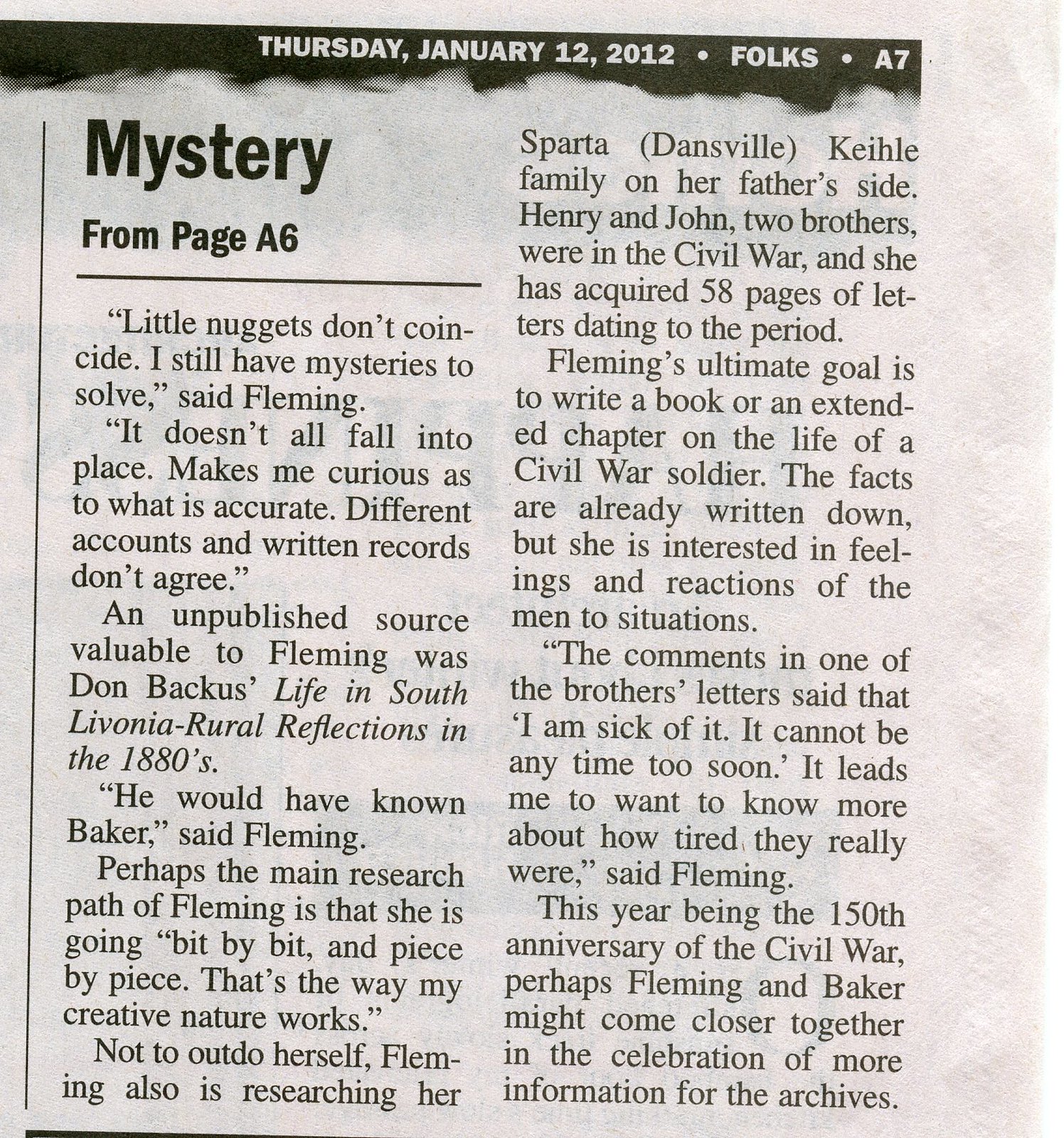The newspaper clipping from Thursday, January 12, 2012, features an article on page A7 with a prominent black strip along the top edge where the date and section information are presented in white text. Below it, the article titled "Mystery from page A6" delves into ongoing historical research. The main subject, Fleming, emphasizes the complexities and discrepancies in historical records, mentioning that "little nuggets don’t coincide." She discusses her curiosity about accuracy, given that different accounts and written records often disagree.

A significant source for Fleming's research was Don Backus’s unpublished work "Life in South Livonia: Rural Reflections in the 1880s," which connected to Baker, a historical figure of interest. Fleming’s meticulous approach to research involves piecing together information bit by bit.

In addition to her primary focus, Fleming is also exploring her own family history, particularly the Sparta, Dansville, and Keele family lineage on her father’s side. She discovered that two brothers, Henry and John, served in the Civil War and has acquired 58 pages of their letters from that period.

Fleming aims to write a comprehensive book or an extended chapter on the experiences of Civil War soldiers, concentrating not just on documented facts but also on the emotional responses and reactions of the soldiers to their circumstances. A poignant quote from one of the brothers, "I am sick of it. It cannot be any time soon," evokes Fleming’s desire to understand the depth of their weariness.

The article concludes with a nod to the significance of the year, marking the 150th anniversary of the Civil War, suggesting that this milestone may bring Fleming and Baker closer to preserving more detailed historical information in the archives.